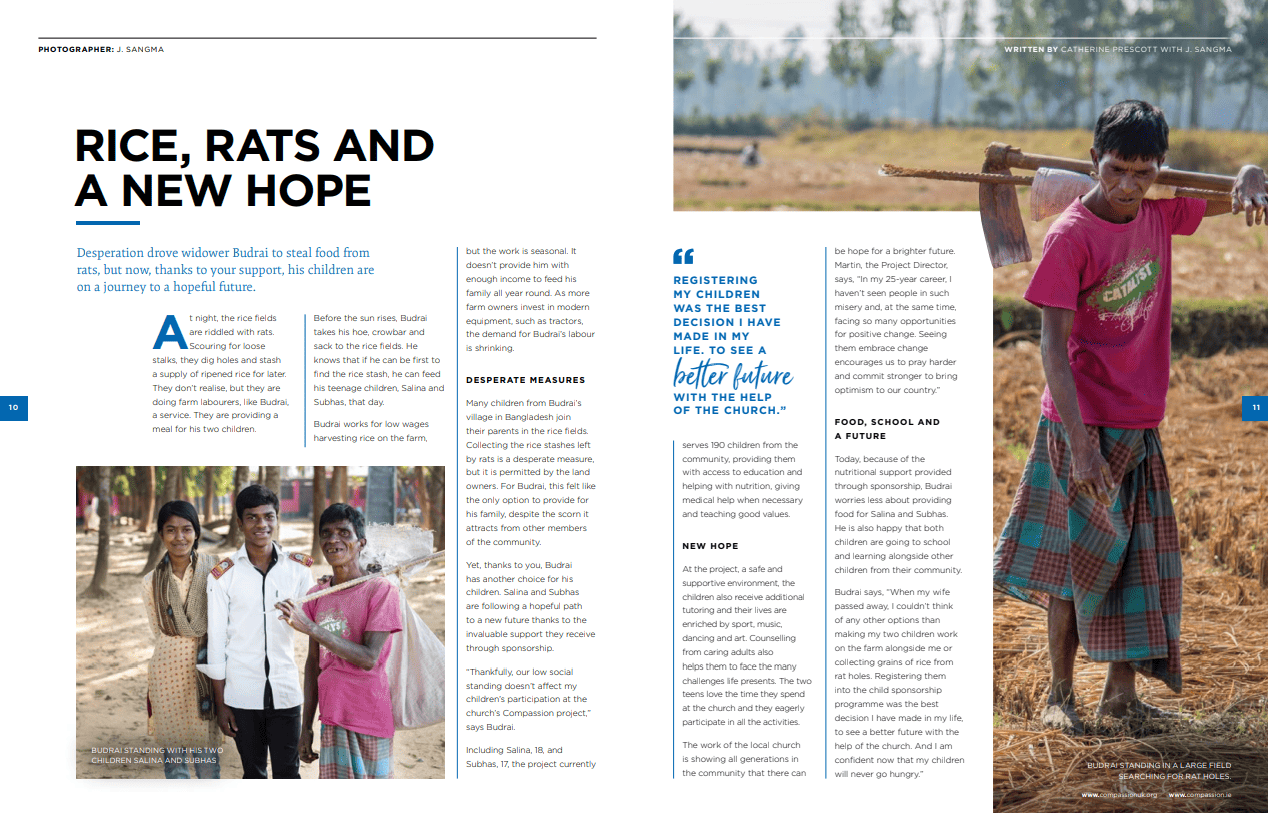This image features a two-page magazine spread. On the left page, at the top left corner, there's a byline that reads, "Photographer Jay Sonoma." Below this, in large, bold black letters, is the headline "Rice Rats and a New Hope." A small blue horizontal line separates the headline from a blue text caption which reads, "Desperation drove widower Bud Ray to steal food from rats, but now thanks to your support, his children are on a journey to a hopeful future." The rest of the left page contains paragraphs that are too small to read clearly.

The focal point of the spread shows an image of three individuals standing in a barren, dirt area with sparse trees in the background. One of the individuals carries a stick with a bag tied at the end, slung over their shoulder. Their clothing and surroundings suggest they come from a region like India or Bangladesh, and they appear to be living in poverty.

Above the image, there's a header titled "Desperate Measures." On the right page, a prominent blue quote says, "Registering my children was the best decision I have made in my life to see a better future with the help of the church." Below this quote, there is a paragraph followed by the subheading "New Hope," then additional paragraphs which appear to provide more details.